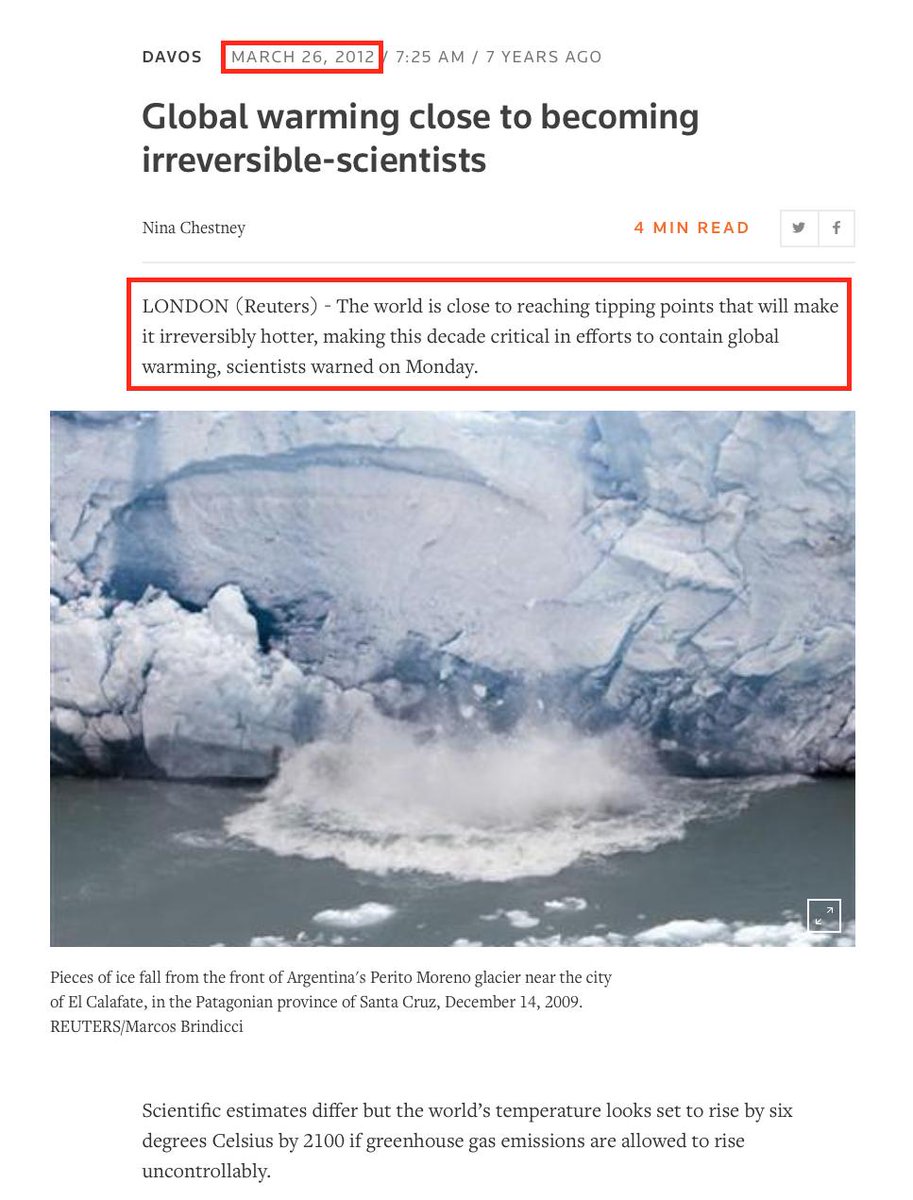**Caption:**

At the top of the image, the word "DAVOS" is prominently displayed in uppercase letters, flanked by the date "March 26, 2012," all within a red-bordered horizontal rectangle. The timestamp reads "7:25 AM," indicating it was taken seven years ago. The article's title, "Global Warming, Close to Becoming Irreversible-Scientists," is written in bold black font, authored by Nina Chesney.

To the right, in a distinct yellow font, the text reads "4 MIN READ" alongside icons for Facebook and Twitter. Another segment enclosed in a red horizontal rectangle states in black text, "London (Reuters)." It highlights the scientists' warning on Monday that the world is nearing critical tipping points, risking irreversible temperature increases and emphasizing the importance of this decade's efforts to combat global warming.

Beneath this, a horizontal rectangular image depicts an iceberg, with pieces of ice visibly falling into the ocean, creating foamy waves. The accompanying caption in small black text reads, "Pieces of ice fall from the front of Argentina's Perito Moreno Glacier near the city of El Calafate in the Patagonian province of Santa Cruz, December 14, 2009." Below, additional text explains that scientific estimates vary, but projections indicate a potential rise in global temperatures by 6 degrees Celsius by 2100 if greenhouse gas emissions continue unchecked.